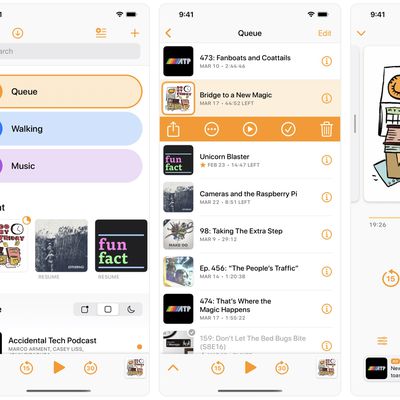The image contains a collage of three screenshots from a mobile music app displayed on a white background. The first screenshot on the left is slightly cut off, about one-eighth of its width. It shows the app's interface featuring buttons labeled "Cue," "Walking," and "Music" at the top. Below these buttons, there are several tiles displaying album covers. At the bottom of this screenshot, one can see playback controls which include a play button, and buttons for fast-forwarding and rewinding by 30 seconds.

The central screenshot is fully visible and shows that the "Cue" section has been selected. This section displays a long list of queued items, each with the album name centered, album artwork on the left side, and an information icon to the right. Additional icons, including a trash can for deletion and a share icon, are visible when interacting with individual album items.

The right screenshot is mostly cut off, showing only about one-quarter of the display. This section seems to mirror the left screenshot's layout with similar playback controls and potentially similar content not fully visible.